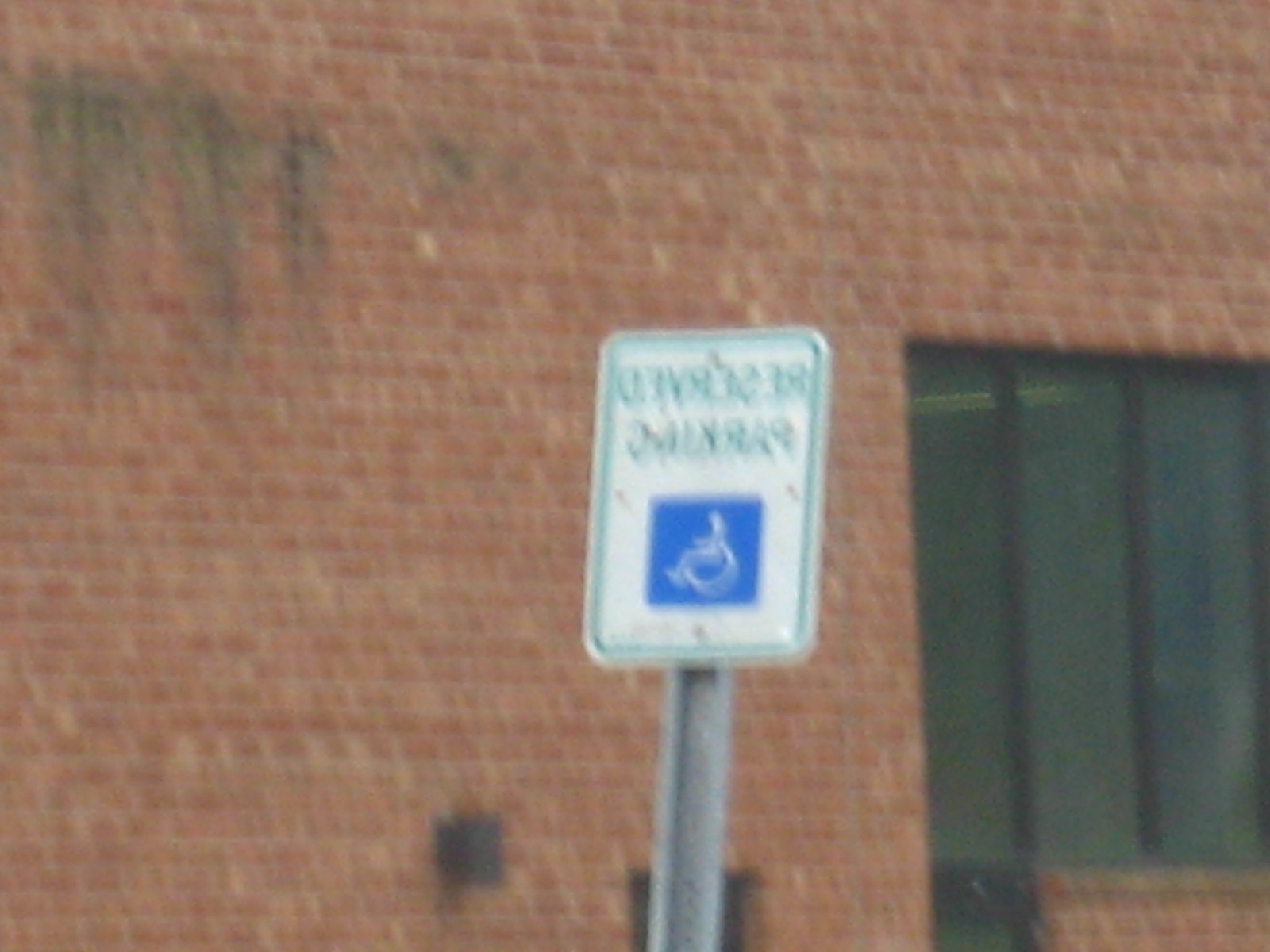This color photograph, though blurred, captures an outdoor scene. The focal point is a small rectangular sign mounted on a metal pole at the center of the image. The sign has a white background bordered by a green rim and features green text, which is not in English and is difficult to read due to the blur. At the center of the sign is a square icon depicting a white wheelchair, indicating accessibility, likely for parking or entry.

In the background, there is a building constructed of small red bricks. Visible toward the right is a window characterized by dark, reflective panes running vertically, suggesting a possible fluorescent light inside the room. The brick wall continues beneath this window, but there is a noticeable gap on the far left side of the wall, filled by a greyish patch instead of bricks. Additionally, there is noticeable discoloration at the top left corner of the wall, showing dark brown or black stains.